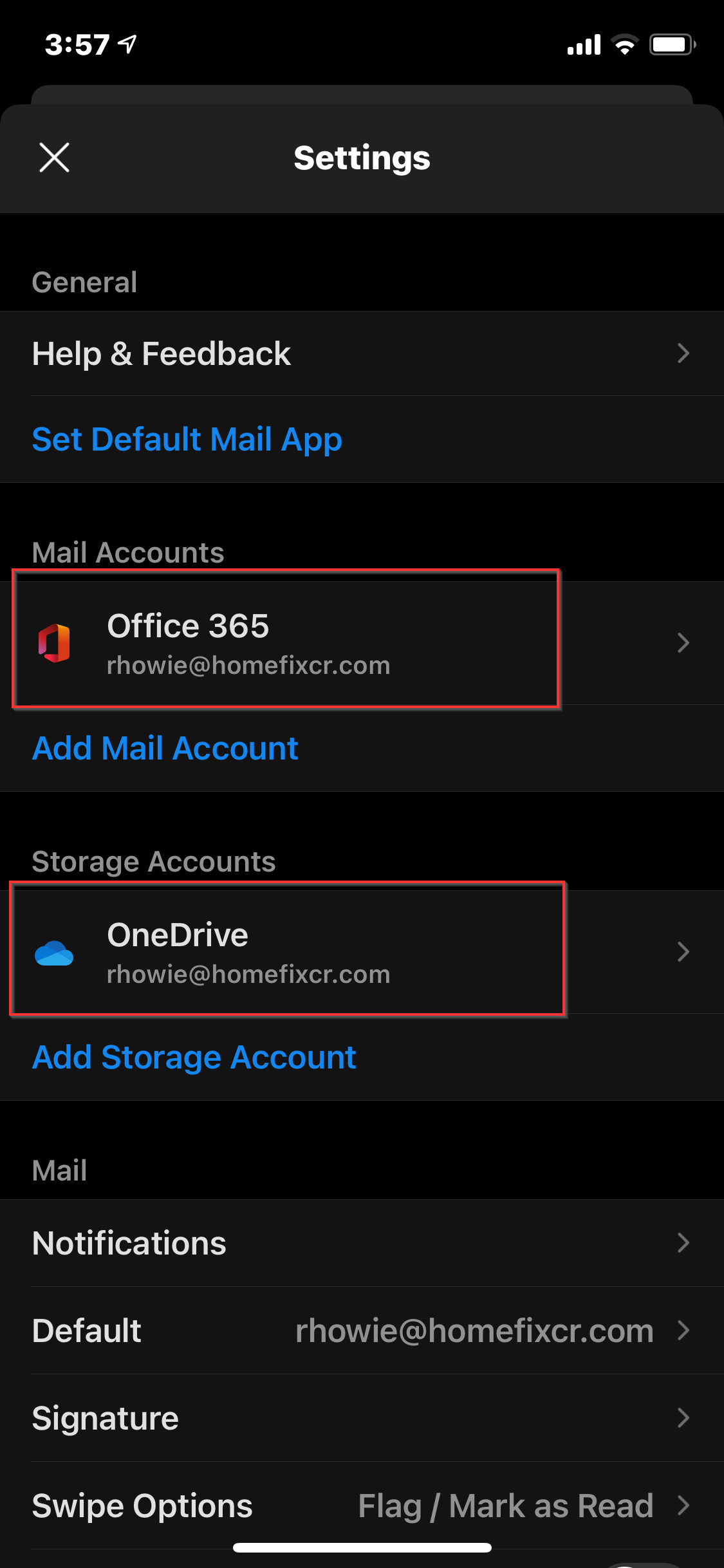The image is a screenshot of a smartphone displaying the "Settings" menu in a vertical format. The background is predominantly black. At the very top left corner, the time "3:57" is displayed along with a small arrow icon. On the top right, the status icons for battery charge and Wi-Fi signal are visible.

The word "Settings" is prominently shown in white text near the top center with a white arrow to its left. Below "Settings" is the section labeled "General." Following this, there are two highlighted boxes: the first one reads "Help and Feedback" in white text, and the second one has "Set Default Mail App" in blue text.

Further down, the "Mail Accounts" section is highlighted with a red rectangular outline. Inside this section, it lists "Office 365" with the Office logo to its left. Adjacent to this, the email address "ourhowie@homefixcr.com" is displayed alongside an arrow icon. Below this, there's an option in blue text to "Add Mail Account."

Subsequently, the "Storage Accounts" section also has a red rectangular outline. It lists "OneDrive" with a cloud icon and the email address "ourhowie@homefixcr.com" next to it. Below this, the text reads "Add Storage Account" in blue.

Finally, the "Mail Notifications" section is mentioned, which shows the same email address, along with options for "Signature" and "Swipe Options," specifying "Flagged/Mark as Read."